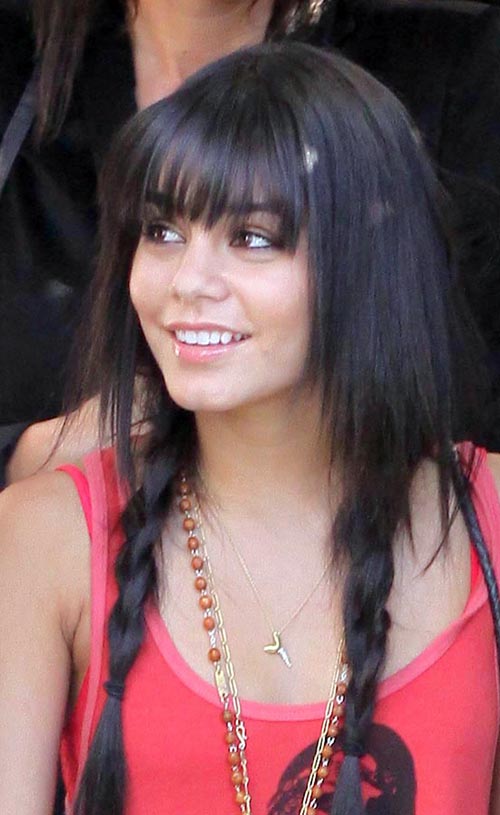This vibrant color photograph captures a young actress with striking dark brown or black hair, styled with the bottom sections in neat French braids that drape over her chest. She has expressive brown eyes and a warm, open-mouthed smile showcasing her bright white teeth. The actress is adorned in a salmon-colored tank top, complemented by multiple gold necklaces, some adorned with orange beads. She exudes a cheerful demeanor, seemingly delighted to be in front of the camera. Although she might resemble Vanessa Hudgens or the actress who played Wednesday in the recent show, her identity isn’t definitively clear from this image. There's a slight hint of someone behind her, but they remain indistinguishable.